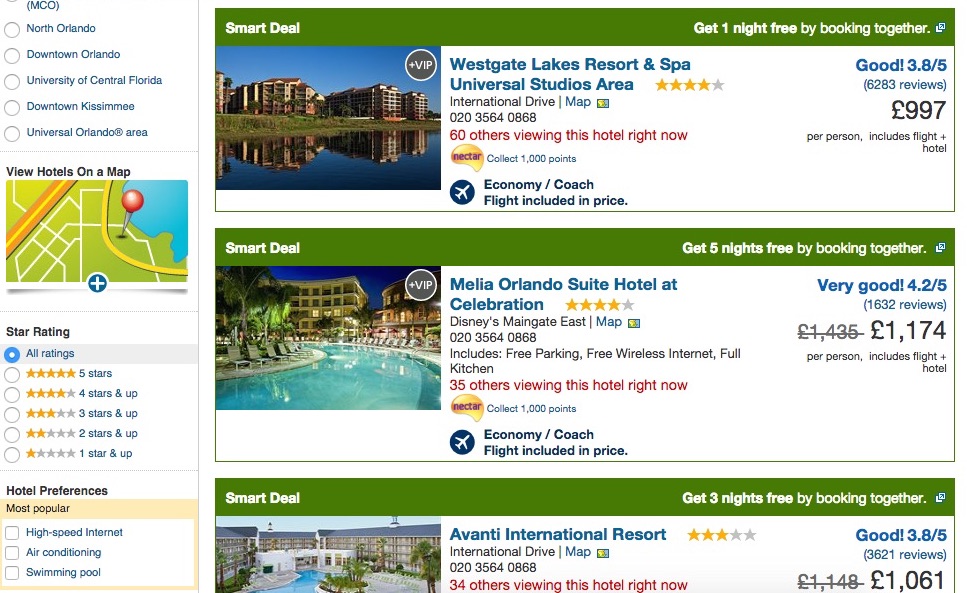The image depicts a holiday booking website with a detailed interface for selecting and booking hotels. On the left-hand side, there is a navigational menu listing areas such as North Orlando, Downtown Orlando, University of Central Florida, Downtown Kissimmee, and Universal Orlando. Additionally, there are options to view hotels on a map and filter search results by ratings, hotel preferences, high-speed internet, air conditioning, and swimming pools.

On the right-hand side of the website, there are promotional deals, highlighted with green banners labeled "Smart Deal." The top deal advertises "Get one night free by booking together" at the Westgate Lakes Resorts and Spa in the Universal Studios area. This hotel boasts a four-star rating with a "Good" score of 3.8 out of 5 based on 6,283 reviews. The price for this package, including flight and hotel, is £997 per person. Additional details include 60 people currently viewing this offer, the opportunity to collect 1,000 points, and an economy or coach flight included in the price.

The second deal features Malaya Orlando Suite Hotel at Celebration, with an image of a swimming pool on the left. This offer provides "Get five nights free by booking together" and has a four-star rating with a "Very Good" score of 4.2 out of 5 from 1,632 reviews. The price is reduced from £1,435 to £1,174 and includes free parking, free wireless internet, and a full kitchen. There are 35 people currently viewing this hotel, with an economy or coach flight included in the price.

The third deal, only partially visible, promotes "Get three nights free by booking together" at Savanti International Resort on International Drive. This hotel also has a four-star rating and a "Good" score of 3.8 out of 5. The price for this package is £1,061, down from £1,148, with 34 people currently viewing the offer. 

Each hotel deal includes comprehensive details such as images, rates, reviews, and special offers, all aimed to help potential customers make informed booking decisions.